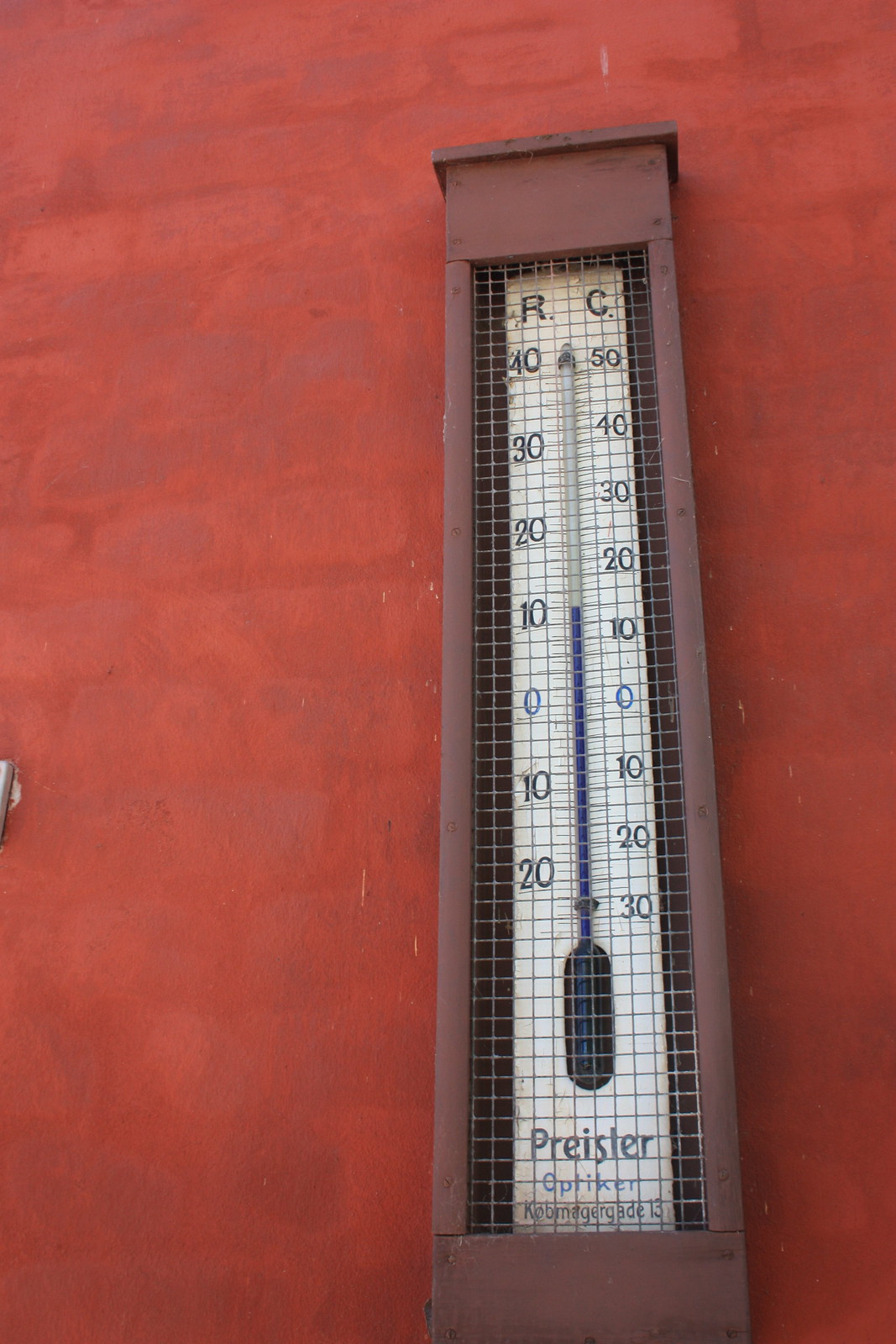This photograph features an antique thermometer encased in a vertically oriented, dark wooden frame. The device is protected by metal wiring within a rectangular wooden box. The background is a deep red hue, giving the impression of red bricks, though the texture is not distinctly brick-like.

The thermometer itself has an off-white backdrop and is marked with two columns; the left column, marked with an 'R' in the top left corner, displays the numbers 40, 30, 20, 10, 0, -10, -20. The right column, marked with a 'C' in the top right corner, shows the numbers 50, 40, 30, 20, 10, 0, -10, -20, -30. A slim glass tube containing blue liquid runs between these columns, indicating a temperature reading just above 10 degrees on the 'R' scale and between 10 and 20 degrees on the 'C' scale. 

At the bottom of the thermometer, there is an inscription that reads: "Pricelar Optiker Kov Mag Magurgad 13".